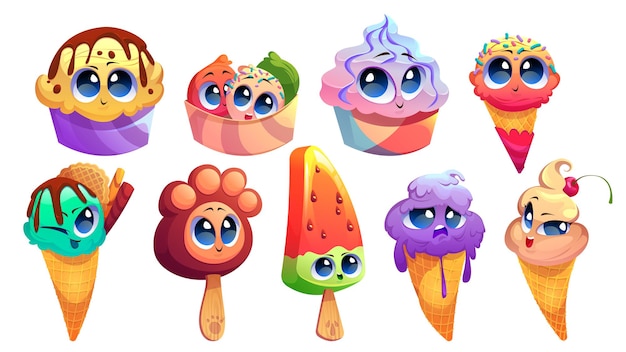The image depicts a charming assortment of cartoon-style ice cream and dessert illustrations, each featuring endearing facial expressions with large, doe-like blue eyes. The vibrant and colorful compositions are meticulously detailed with rich gradients and shadows, making them appear whimsical and lively. Arranged in two rows, the top row consists of four treats: 

1. A yellow ice cream adorned with brown sauce, set in a round purple bowl.
2. A striped orange cup holding two scoops of peach ice cream with a decorative leaf.
3. A swirled pink and purple soft serve in a vividly colorful bowl.
4. A cone of orange and yellow ice cream sprinkled with red, yellow, and orange accents.

The bottom row includes five unique ice creams:

1. A waffle cone filled with peach ice cream resembling whipped cream, topped with a maraschino cherry.
2. A purple ice cream cone dripping with charm.
3. A watermelon-shaped ice pop on a stick, complete with seed details.
4. A paw-shaped ice pop with a playful expression.
5. A green ice cream in a waffle cone, accented with brown sauce and two stick-like wafers or cinnamon sticks.

Each dessert character is unique yet unified by their similar expressive eyes and small mouths, creating a delightful and cohesive visual feast.